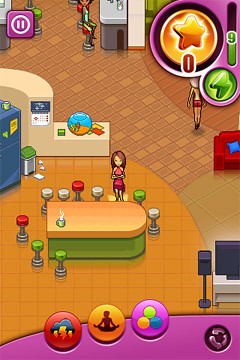This image appears to be a vibrant, colorized screenshot from an old-school video game, likely designed for an early computer or classic mobile device. The setting is a detailed, nostalgic virtual kitchen. The kitchen features a yellow-gold tiled floor and a prominently placed U-shaped table with a wooden top and green base. The table is surrounded by an assortment of barstool seats in alternating colors: white, green, white, and red. A cartoon-like avatar, characterized by her brown hair and pink dress, stands outside the perimeter of the table, adding a touch of charm to the scene.

In the backdrop, typical kitchen elements such as a refrigerator, countertop, and a calendar are visible, enhancing the realism of this virtual space. Through the game's pixelated graphics, other rooms are faintly discernible in the distance, although they lack the clarity and detail of the kitchen area. This richly detailed scene captures the essence of classic gaming nostalgia, blending an everyday setting with vintage digital artistry.